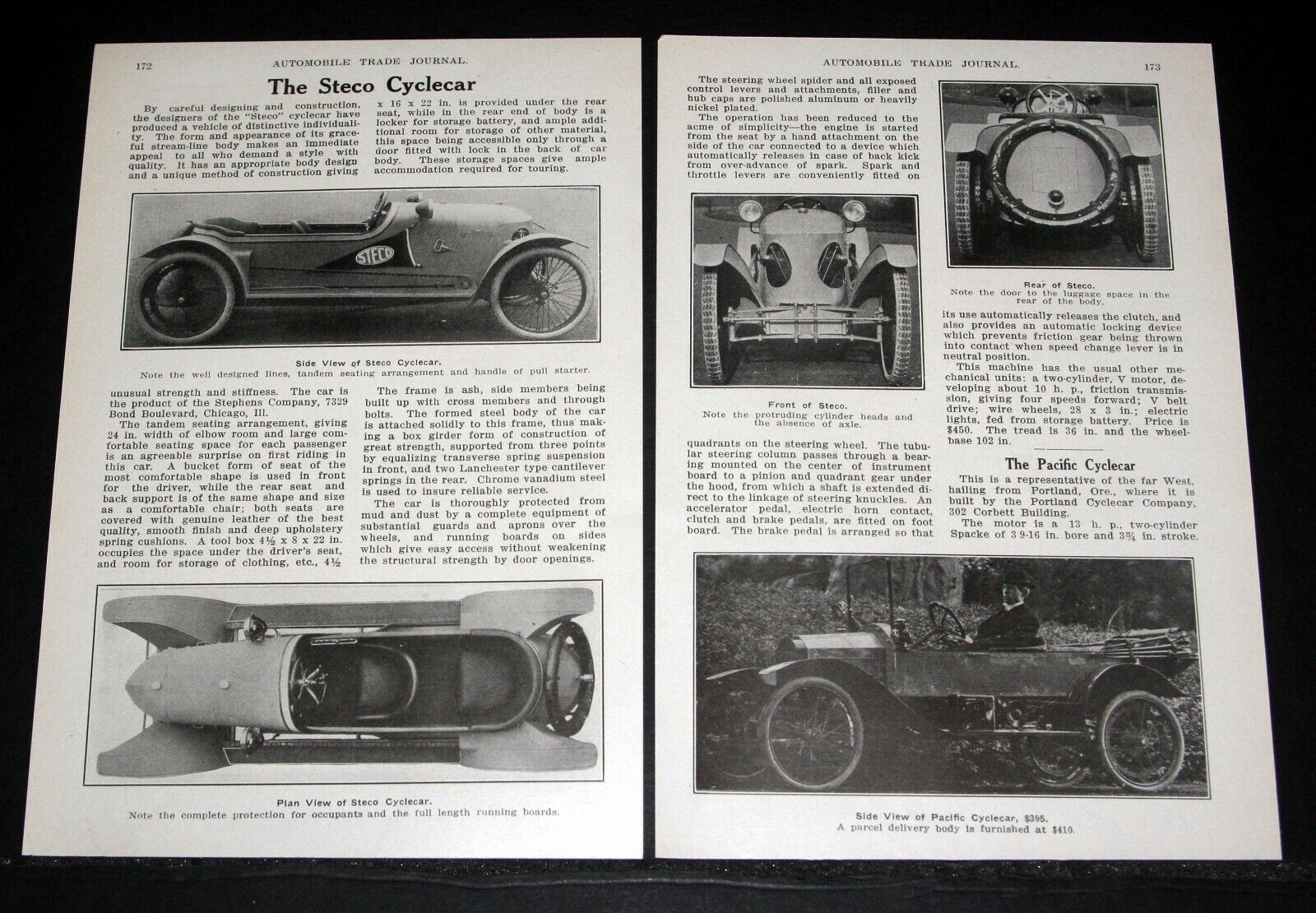The photograph captures a vintage, possibly shellac or plastic-coated magazine or pamphlet spread open, revealing two pages filled with detailed information about antique automobiles. The left-hand page is titled "The Steko Cycle Car" in a classic typeface resembling Times New Roman, although the text beneath the title is too small to read clearly. This page features two black-and-white photographs of a cycle car: a side view showcasing its bicycle-like tires and a simple, dark-colored body similar to a child's pedal car, and a top view that reveals the car's two-seater configuration, with a front seat for the driver and a rear seat for the passenger, along with a spare tire mounted on the back.

The right-hand page, which seems to be part of the "Automobile Trade Journal," contains three black-and-white images of another cycle car version known as the Pacific cycle car. The first photo captures the front view, where the car's headlights and spoke wheels are visible. The second image displays the car's rear, complete with a spare tire on its trunk. The final picture depicts a man wearing a derby hat, seated at the steering wheel of the antique car, with a rustic, wooded backdrop behind him. The images and text evoke a nostalgic glimpse into early 20th-century automotive design.